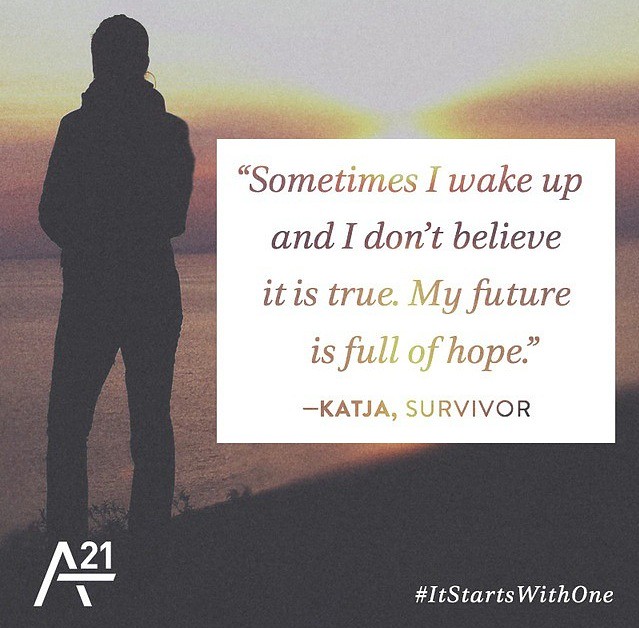The image is a square photo with a detailed background and an inspirational quote in the center. Dominated by shades of gray with hints of yellow and orange reminiscent of a sunset, it features a silhouette of a person standing on a cliff, looking out over a brownish body of water, and a shadowy black hill. The colors blend in a somewhat blurry, dreamy fashion, creating an emotive and reflective atmosphere.

Central to the image is a large white square containing a poignant quote from Katja, a survivor. The text reads, "Sometimes I wake up and I don't believe it is true. My future is full of hope." This quote overlays the background so that the sunset's colors subtly come through.

At the bottom of the image, additional text elements provide context. On the lower left, white text reads "A21," likely signifying the organization or initiative behind the message. In the lower right, in white italics, is the hashtag "#ItStartsWithOne," adding a call to action or campaign slogan to the visual narrative. Overall, the image combines elements of hope and resilience with a visually striking sunset setting.